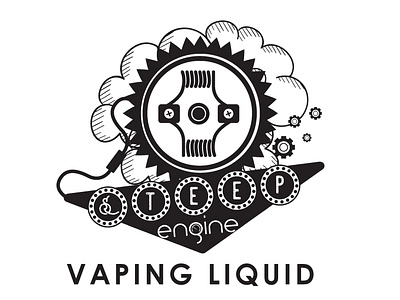This is a grayscale business logo for a vaping liquid brand named "Steep Engine." The central design features a circular element resembling a mechanical engine, surrounded by jagged, spiky ridges that further emphasize its industrial theme. Behind this engine symbol, there is a cloud which seems to be connected by a cord. Below this, a wide black triangle suggests the shape of an electric light-up sign, and inside, it spells out "STEEP ENGINE." Each letter of "STEEP" is individually circled. Below this triangle, the text "VAPING LIQUID" is prominently displayed. Additional mechanical parts and abstract designs in the background add complexity to the graphic, enhancing the industrial and mechanical aesthetic of the logo.